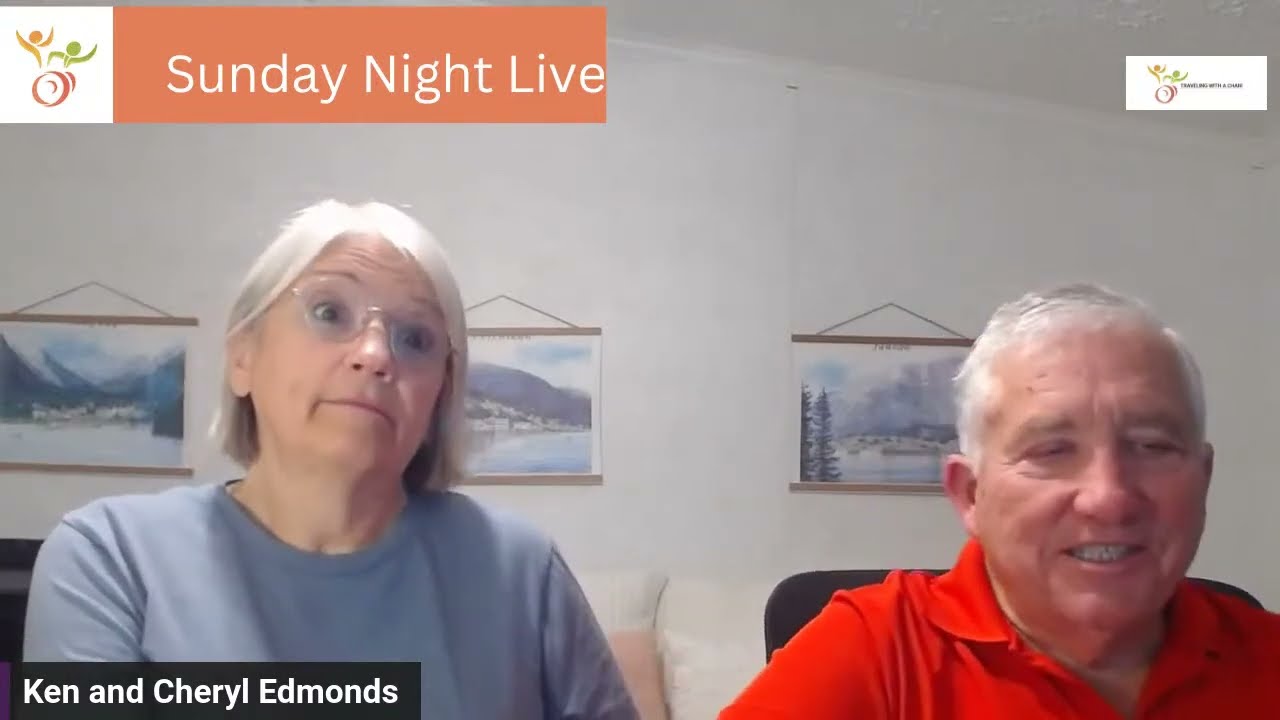This image is a screenshot from a webcam, capturing an older couple identified as Ken and Cheryl Edmonds. They appear to be in their late 60s or early 70s. The woman, seated on the left, has shoulder-length, solid gray hair, and wears thin wired glasses along with a periwinkle blue long-sleeve shirt. She displays a straight mouth and raised eyebrows, giving her a slightly surprised expression. To her right sits Ken, who sports gray swept-over hair and a red polo shirt. He has a round, bulbous nose and a half-smile that reveals his teeth. The background features a white wall adorned with three small scenic paintings. At the top left corner of the image, there is text with an orange background that reads "Saturday Night Live." The bottom left corner introduces the couple with the text "Ken and Cheryl Edmonds" in white font on a black box.